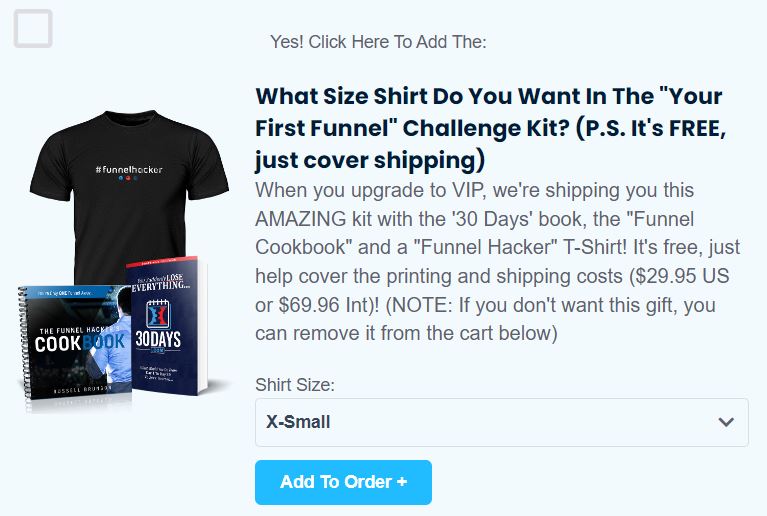Here is a cleaned-up, detailed caption:

---

This is an advertisement or an order page for a special t-shirt offer. In the upper left corner of the image, there is a gray square. Centrally positioned on the page, there is a vibrant call-to-action blurb that reads "Yes! Click here to add:", encouraging users to engage with the content. Below this text, in a distinctive Bladger font, a question prompts, "What size shirt do you want in the 'Your First Funnel' Challenge Kit?"

A smaller aside in parentheses reads: "P.S., it's free, just covering shipping," clarifying the terms of the offer. The message continues: "When you upgrade to VIP, we're shipping you this amazing kit which includes the '30 Days' book, 'The Funnel Cookbook,' and a 'Funnel Hacker' t-shirt. It's free; just help cover the printing and shipping costs—$29.95 U.S. or $69.96 international."

---

This revised caption provides a clear and thorough description of the advertisement while organizing the details coherently.